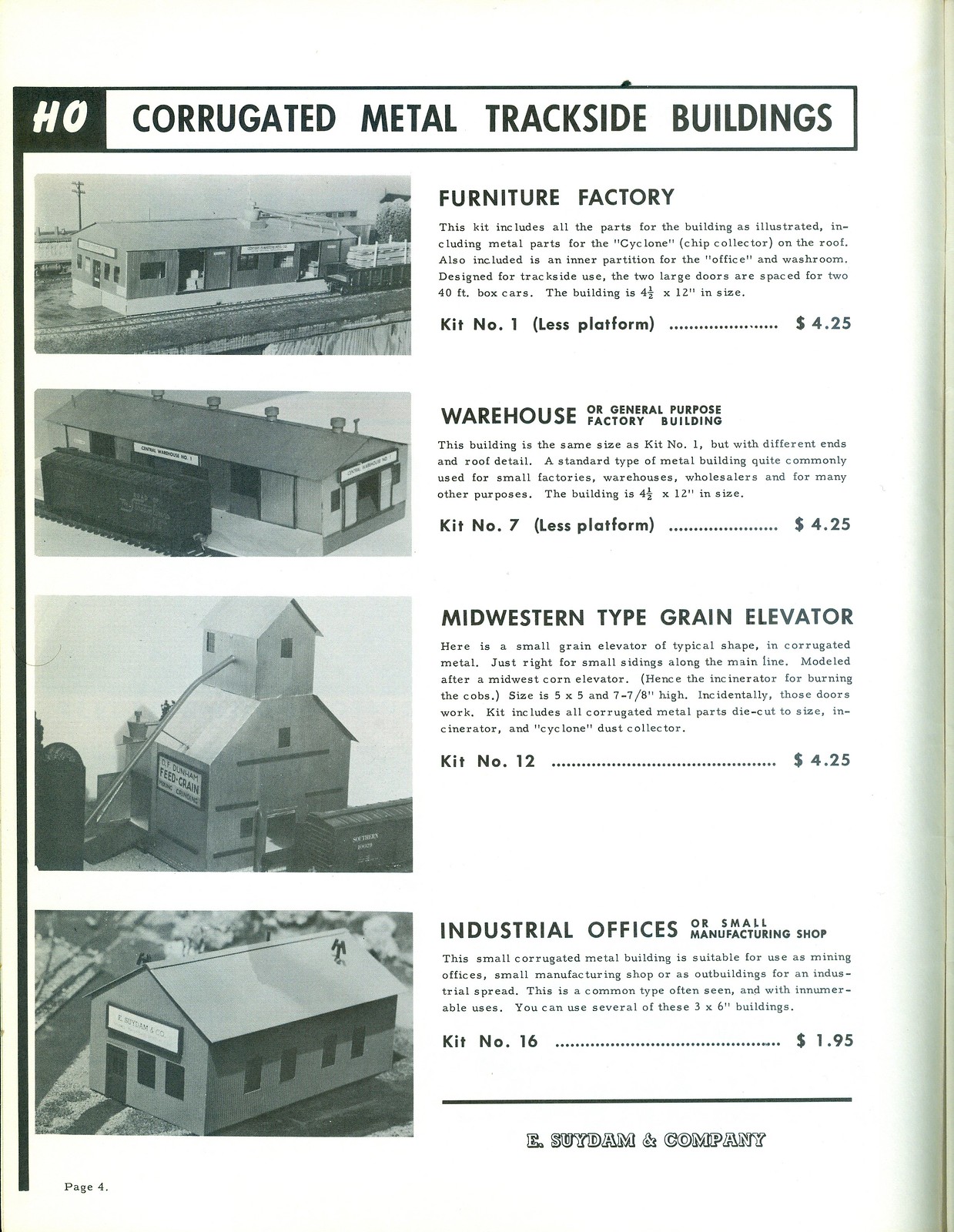This scanned image, resembling a page from a catalog or magazine, showcases a listing of HO scale model buildings intended for train sets. The paper is light gray, darkening toward the right edge. The top of the image features a black-bordered white rectangle with the text "Corrugated Metal Trackside Buildings" in bold, black, all-capital letters, alongside a black square with white "HO" lettering. Below this header, the left side of the page displays four stacked black-and-white photographs of individual industrial buildings. Each building, depicted in the photographs, is accompanied by a detailed description and pricing on the right side of the page in bold text. The buildings are titled: "Furniture Factory," "Warehouse or General Purpose Factory Building," "Midwestern Type Grain Elevator," and "Industrial Offices or Small Manufacturing Shop." Descriptions specify included parts, dimensions, and kit numbers, with prices listed—$4.25 for the first three buildings and $1.95 for the fourth.